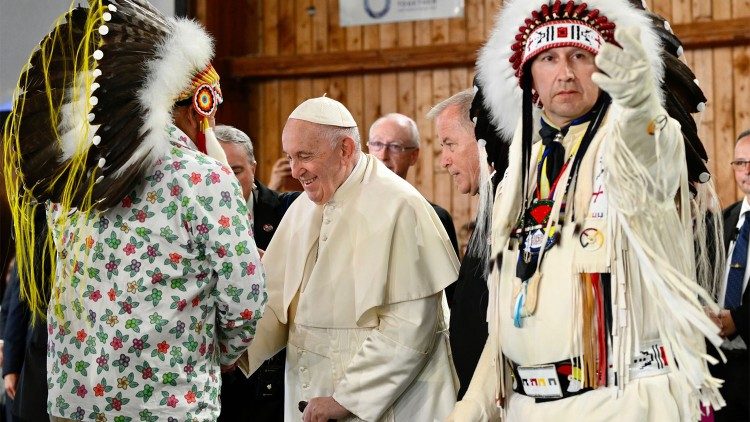In a large room with predominantly wooden walls, an image captures Pope Francis, dressed in his traditional white robe and skull cap, smiling warmly as he shakes hands. Flanking him are two men adorned in intricate Native American attire. The man to his right wears a cream-colored outfit embellished with long leather fringes on the sleeves, gloves, and a grand feather headdress. The man to his left has his back turned, showcasing a black feather headdress accented with white feathers. Surrounding this central trio are several men in dark suits, adding a formal backdrop to the culturally diverse foreground. The Pope appears to be the focal point, with the gesture of greeting underscored by the vibrant and symbolic Native American garments.